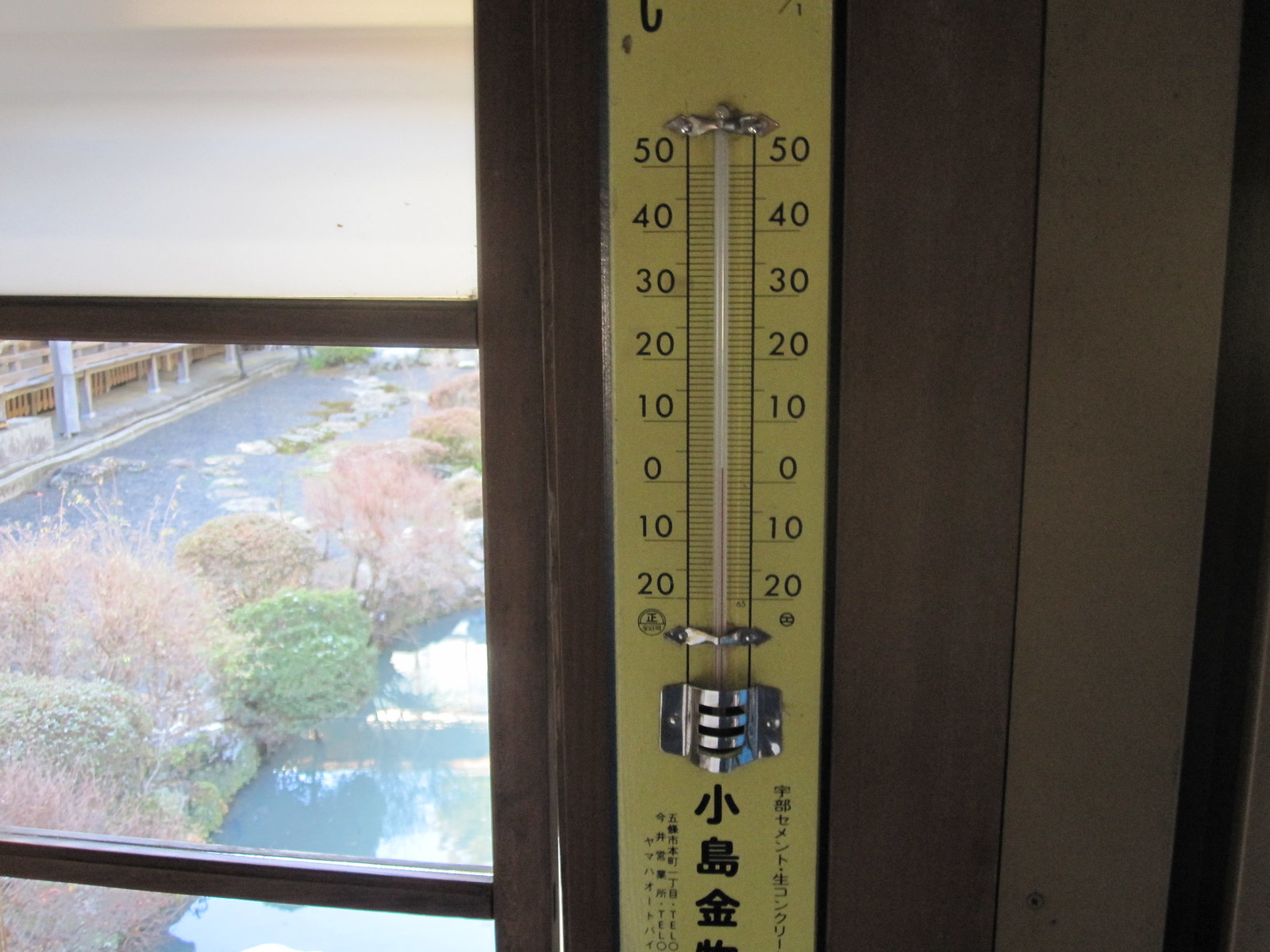In this image, a yellow-backed thermometer, mounted on a brown wall, is situated beside a window that offers a view of a lush outdoor area. The temperature gauge, characterized by its dual scale ranging from 20 to 50 on both the left and right sides, features a visibly red indicator hovering around the 4 mark. The thermometer is secured with three chrome rings and includes some vertical Asian script, possibly Japanese or Chinese, at its base. The window reveals a landscape of short trees adorned with a mixture of green and red foliage, suggesting an elevated perspective from the third or fourth story of the building. The top portion of the thermometer faintly displays the letter "C," hinting at the measurement unit, although it remains indistinct.